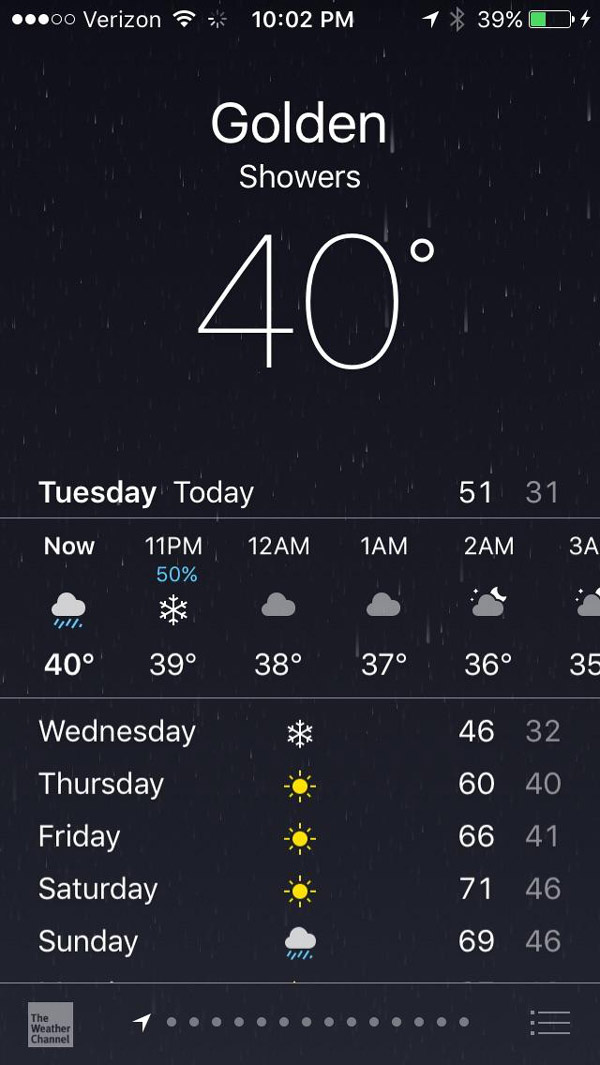A grayscale screenshot displays the screen of a mobile device, possibly a phone or tablet, with a predominantly black background punctuated by scattered grey dots. The top bar indicates it is connected to Verizon's network, with Wi-Fi enabled, Bluetooth turned off, and the battery level at 39%. The time displayed is 10:02 PM.

The screenshot seems to reflect weather information for a location named Golden. At 10:02 PM, the temperature is 40 degrees Fahrenheit, with a forecast of showers. The weather details for the upcoming hours are as follows: at 11 PM, it will be 40 degrees, cloudy, and raining, with a 50% chance of snow. From midnight to 2 AM, the forecast shows cloudy conditions with light precipitation.

The extended forecast for the rest of the week indicates varying weather patterns. On Wednesday, snow is anticipated, followed by sunny days on Thursday, Friday, and Saturday. Rain is expected on Sunday. The high temperatures for the coming days are forecasted as follows: Wednesday at 46°F, Thursday at 60°F, Friday at 66°F, Saturday at 71°F, and Sunday at 69°F.